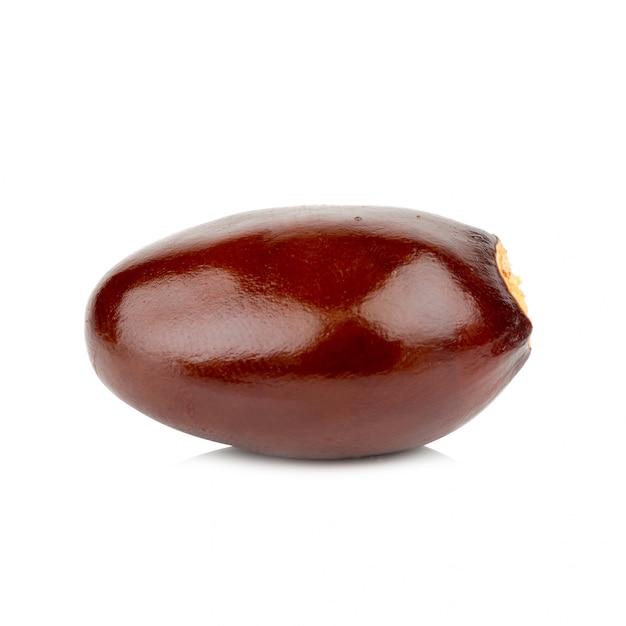The image features a close-up of an oval-shaped brown object set against a stark white background. The item presents a glossy surface with light reflecting off its center, creating a white shine, while a subtle shadow beneath it adds depth. The object seems to be longer on the top than on the sides and has a slightly flatter end, possibly where a stem might have been. One consistent detail among the interpretations is the appearance of a yellowish or orangey section on the right side, which could indicate a removed stem or a bitten-off portion, suggesting it might be a food item. The image is simplistic, devoid of any text, borders, or additional elements.